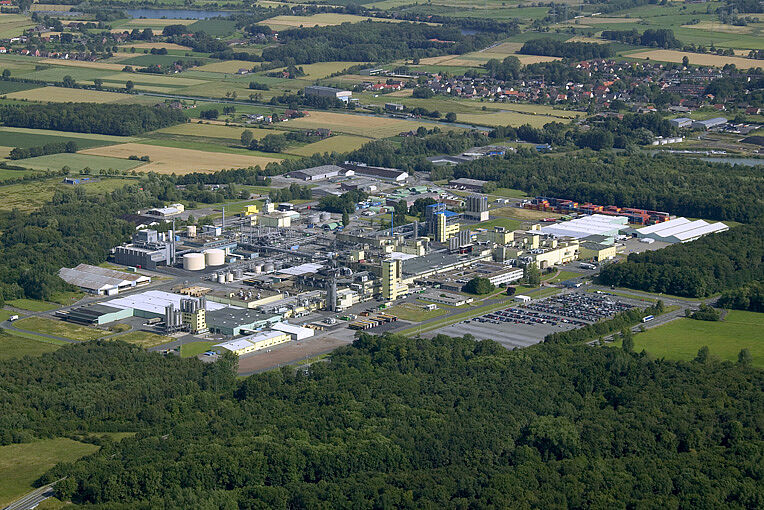An aerial view captures a vast factory complex consisting of multiple industrial buildings in shades of gray and yellow, dotted with machinery and silos, indicating a large power plant or meat processing plant. The expansive complex is encircled by lush green trees with fluffy treetops and sprawling farmland, creating a stark contrast between the industrial site and the surrounding natural landscape. A large parking lot, half-filled with cars, is situated in front of the factory. The image also includes blue, white, red, and patches of bright yellow, adding to the complexity and richness of the scene. In the distance to the left, there's a patch of additional structures that might indicate a rural area, while on the right, there are hints of a more urban setting, possibly a city.